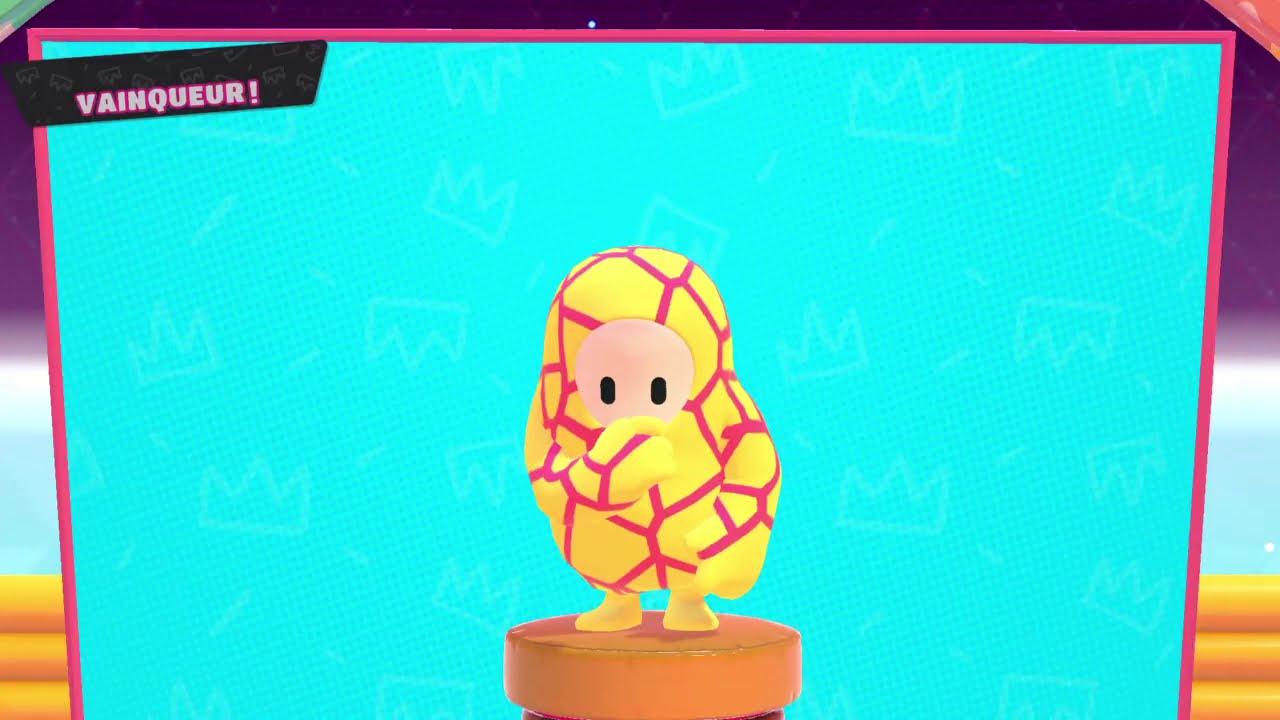This detailed caption describes a screenshot from the video game Fall Guys featuring a victorious character. The central character, resembling a yellow bean or baby chick shape, has intricate red cobweb-like patterns coursing through its body, arms, and head. The character is posing with its right hand in front of its mouth and its left hand down, standing on a brownish-orange podium. The backdrop features an aquamarine blue screen with a thin red border. Additionally, there are inflatable walls in yellow at the bottom corners. In the upper left corner of the screen, the word "Vainqueur!" appears in silvery-gray letters with a red outline atop a pink background, indicating a win. The overall background consists of a purple-black sky with a light blue center.